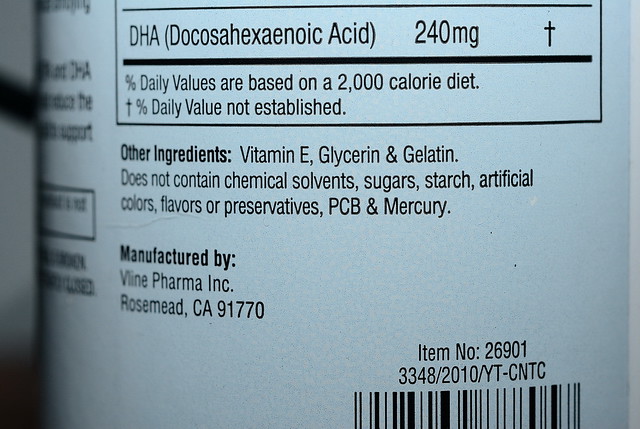This image showcases a nutritional supplement prominently featuring DHA, with a concentration of 240 milligrams per serving. The supplement also includes Vitamin E, glycerin, and gelatin among its ingredients. The label highlights the absence of chemical solvents, sugars, artificial colors, flavors, preservatives, PCB, and mercury, ensuring a cleaner and safer product for consumption. The manufacturer's details appear slightly blurred but suggest "Veline Pharma, Inc." based in Rosemead, California, 91770.